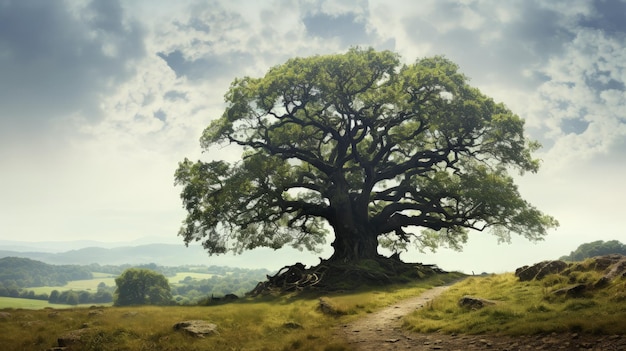This is a photograph of a gnarly, ancient tree perched atop a hillside, serving as the centerpiece of the scenic outdoors. The tree boasts a wide and thick trunk with branches that spread out impressively, winding and curling in a gnarled fashion. Its sturdy, short, yet massive brown trunk supports a dense canopy of lush green foliage. Around the tree, the landscape features rugged stones, small rock outcroppings, and a dirt path that snakes through the scene. Grasslands permeate the hillside, and in the distance, a mixture of hills, some trees, and an outline of mountain ranges add depth to the setting. The sky above is light blue with wispy white clouds, indicating a sunny, albeit slightly cloudy day. The overall atmosphere is serene, encapsulating the timeless beauty of nature.